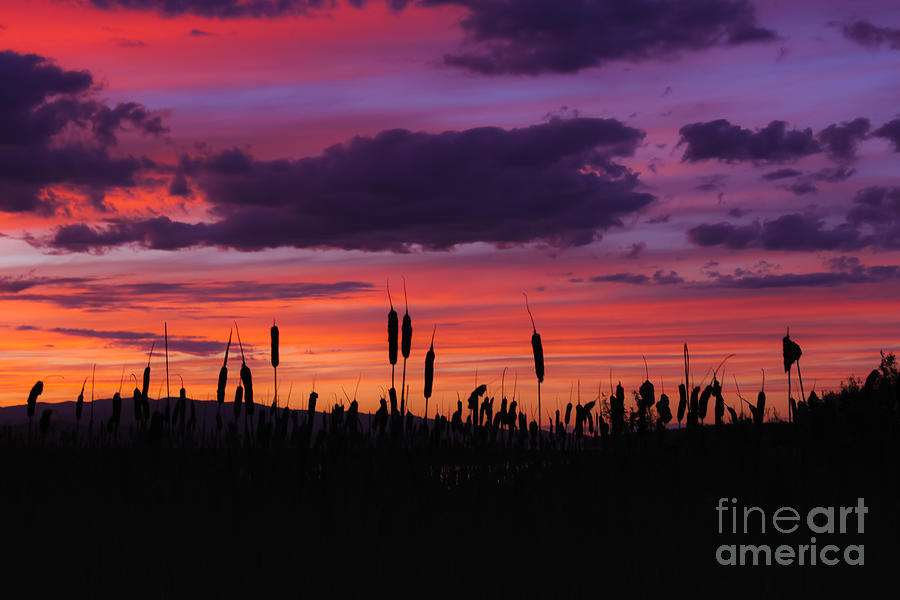A breathtaking photograph captures a vivid sunset over a silhouetted field of cattails or reeds, likely positioned in a swampy area. The foreground is dark, with the plants resembling hot dogs poking up into the scene, creating striking black silhouettes against the vibrant backdrop. The sky exhibits a stunning display of colors, with streaks of red, orange, and yellow near the horizon, transitioning to dark purple and blue hues higher up. Shadowy outlines of mountains can be discerned in the background, adding depth to the image. A discreet "Fine Art America" logo is visible in the bottom right corner of the photo.